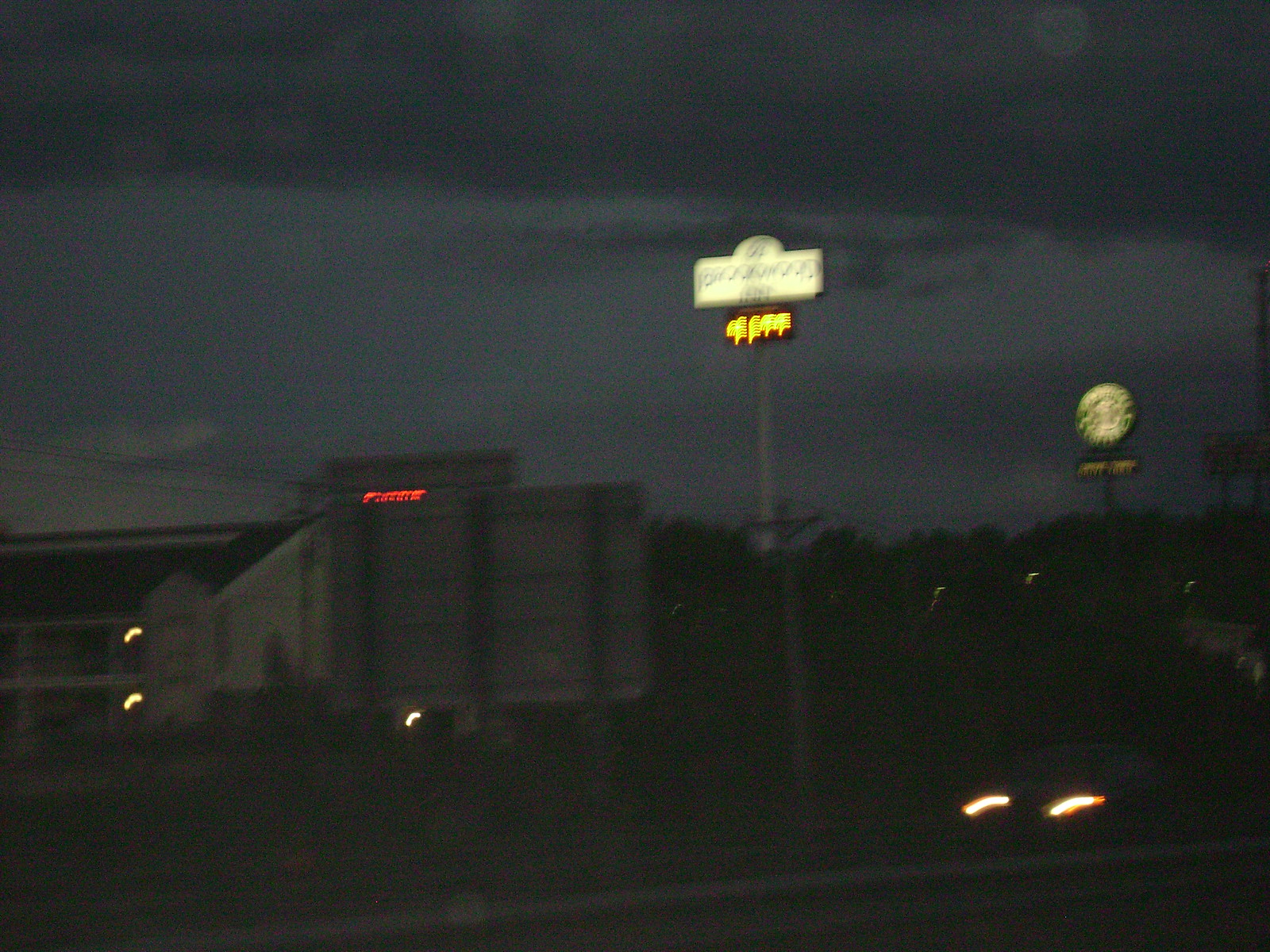This nighttime exterior photograph captures a dynamic and somewhat blurry scene, likely taken from a moving vehicle. In the lower right corner, the image is particularly blurry, adding to the sense of motion. The vehicle's headlights appear as short streaks in the frame, further emphasizing movement. On the left side, the outline of a large, light-colored building is visible, topped with an unreadable red-lit sign, its form softened by the motion blur. Dominating the right side is a very tall, illuminated Starbucks sign, recognizable by its green background and iconic white logo. Centrally positioned, a much taller, horizontally rectangular sign with a slight dome in the middle extends up into the dark, cloud-covered sky. This sign is white with what seems to be black lettering, though its text is not legible due to the blur and lighting conditions. The overall image conveys a sense of motion and the characteristic hustle of a nocturnal urban setting.